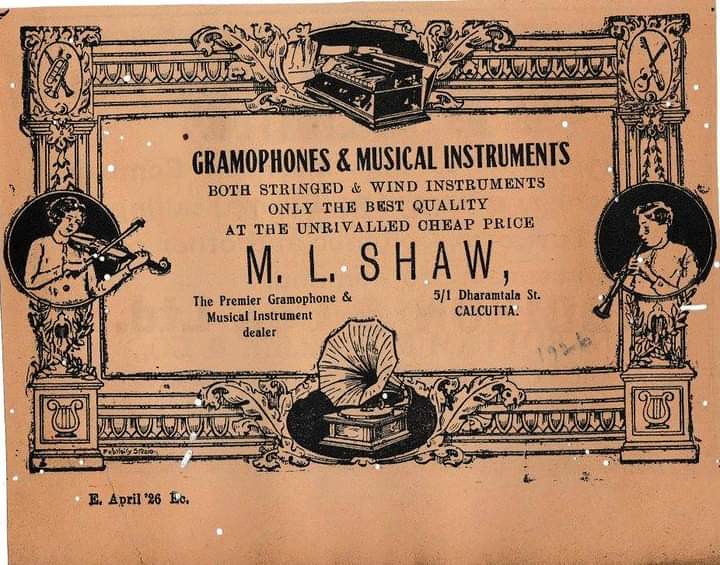This image features an antique rectangular poster, its background aged to a light brown hue speckled with white spots and black smudges. The poster serves as an advertisement for musical instruments, encased in an intricate, black pen-drawn frame wider than it is tall. This ornate border, resembling crown molding, showcases detailed black and white illustrations of various musical instruments and musicians. At the top center, there's a depiction of a piano or organ, while the bottom center features an image of a gramophone with a large speaker. On the left side, a young girl plays the violin, and on the right side, a young boy is depicted with a clarinet.

In the center of the poster, bold black text reads: "Gramophones and musical instruments, both stringed and wind instruments. Only the best quality at the unrivaled cheap price. M.L. Shaw, the premier gramophone and musical instrument dealer, 5/1 Dharmalala Street, Kolkata." Additional drawings of musical instruments are sprinkled around the border, further emphasizing the theme. At the bottom left corner, the text "E. April 26" is inscribed, adding a historical touch to this charming vintage advertisement.